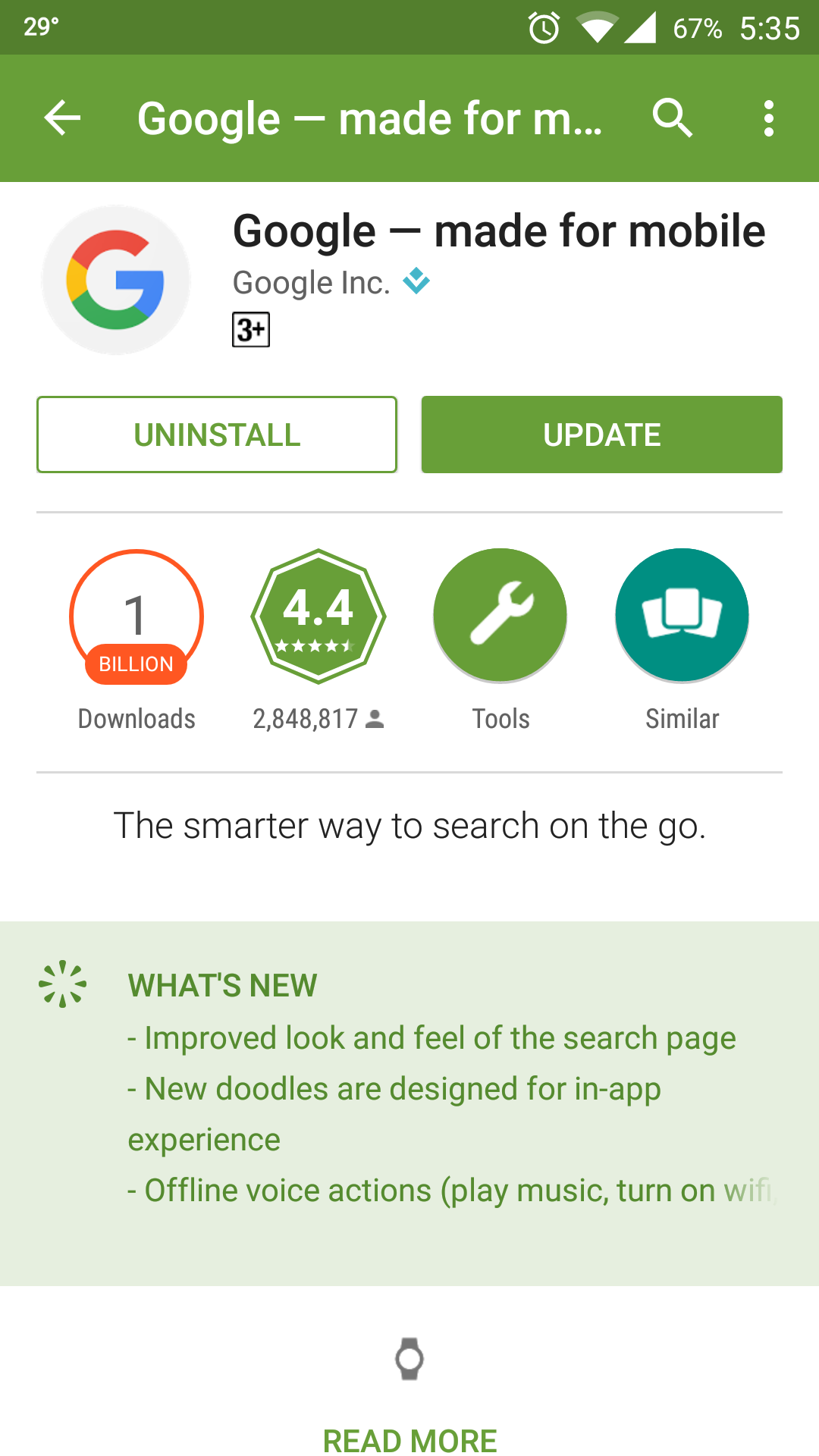The image displays a screenshot of the Google App page within a mobile app store. Dominating the top left is the recognizable Google logo, with the iconic 'G' in red, yellow, green, and blue. The header area at the top of the screen is green and shows various status icons: a temperature of 29 degrees, the time as 5:35, a battery level at 67%, the Wi-Fi symbol, and a clock.

Below this header, there are two buttons: "Uninstall" and "Update." The "Uninstall" button has a white background, while the "Update" button features a green background. Moving further down, the app page indicates that Google has been downloaded 1 billion times, holds a 4.4-star rating, and belongs to a category denoted with a tools icon. Additionally, a teal-colored circle with the word "Similar" is visible.

The description section below highlights that Google is marketed as "the smarter way to search on the go." It also notes recent updates, including an "improved look and feel of the search page." The section wraps up with the prompt to "Read more," inviting users to explore further details.